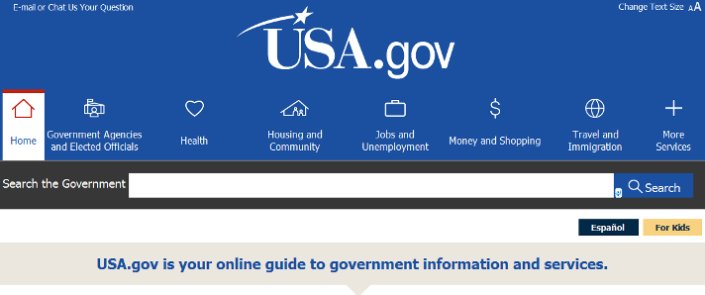Screenshot of USA.gov Desktop Application Interface

This detailed screenshot captures the user interface of the USA.gov desktop application. The background predominantly features shades of blue. At the top left corner, text encourages users to "Email or chat us your question." Centrally located at the top is the USA.gov logo. In the top right corner, a "Change text size" option is available, symbolized by a smaller 'A' and a larger 'A,' both capitalized.

Underneath the header, several tabs are present. The "Home" tab is highlighted against a white background. Adjacent tabs include "Government Agencies and Elected Officials," "Health," "Housing and Community," "Jobs and Unemployment," "Money and Shopping," "Travel and Immigration," and "More Services."

Beneath these tabs, a predominantly black banner features a white text field labeled "Search the Government," paired with a blue search button adorned with a magnifying glass icon.

To the right, two options are available: "En Español," displayed against a black background, and "For Kids," marked by a slightly yellowish-orange rectangle.

Further down, a grayish background supports the text: "USA.gov is your online guide to government information and services." This text serves as the footer and concluding message of the screenshot, encapsulating the service’s purpose.

Overall, the screenshot presents a clean, user-friendly interface designed to facilitate easy access to various government resources and services.